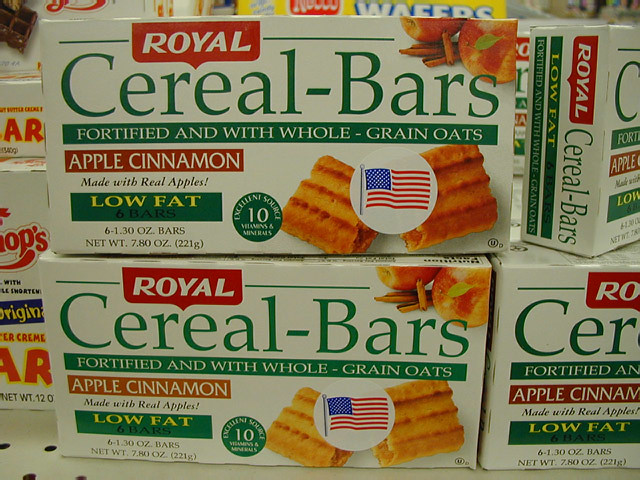Close-up shot of a grocery store shelf stocked with rows of Royal brand cereal bars. The white metal shelving is packed with neatly arranged boxes. Each box is predominantly white, featuring a red banner that reads "Royal." Below, in white letters on a green banner, it states "Cereal-Bars," followed by another green banner proclaiming "Fortified with Whole Grain Oats." Further down, a red banner announces the flavor, "Apple Cinnamon," and emphasizes "Made with Real Apples!" in prominent text. A green banner with yellow lettering highlights the product as "Low Fat." The box also prominently displays an image of a cereal bar cut in half, and a circular emblem above it contains an American flag, indicating the product's origin.